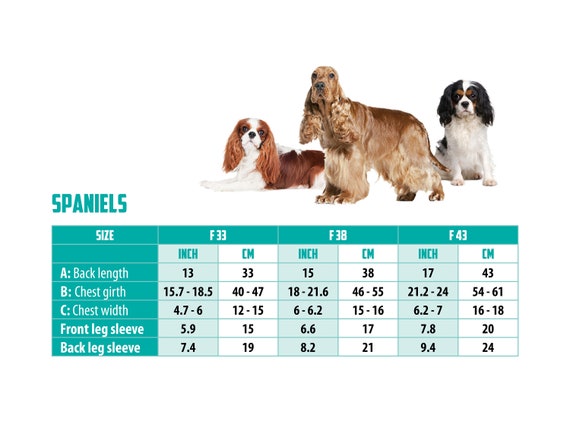The image portrays a detailed graphic design featuring three different Spaniel dogs positioned beneath a teal-colored title reading "Spaniels." On the right side, there's a black, white, and brown tricolor Cocker Spaniel with an alert gaze directed towards the camera. In the middle stands a larger golden tan Cocker Spaniel, distinguished by its long, fluffy ears and sleek, shiny fur, also looking towards the camera. To the left, a Cavalier King Charles Spaniel, characterized by its white coat with dark brown markings and resting posture, looks up towards the camera.

Beneath the trio of dogs is a table extending across the entire width of the image. The table categorizes the dogs based on sizes labeled as F33, F38, and F43, with measurements provided in both inches and centimeters. Each size column specifies the dogs’ back length, chest girth, chest width, front leg sleeve, and back leg sleeve dimensions, offering a comprehensive overview of the physical attributes for each type of Spaniel.